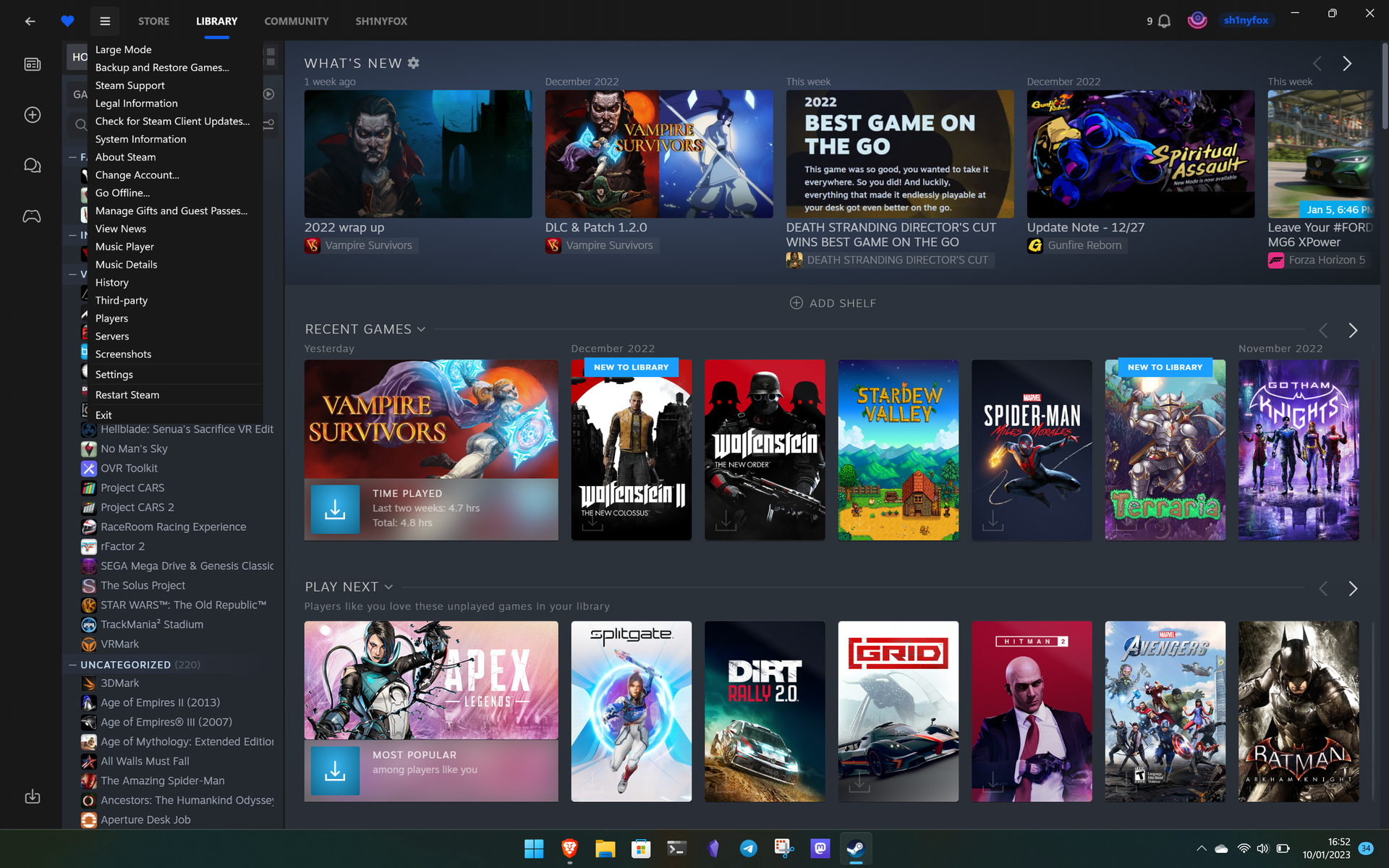The image showcases the main screen of a digital gaming platform, resembling the interface of services like Netflix, set against a black background. At the top, there is a menu bar featuring a blue heart icon for favorites, and labeled options including "Store," "Library," and "Community." 

Beneath this bar, various game icons are displayed in rows. The top row features:
- An image of a zombie-like character with the label "2022 Wrap-Up."
- “Vampire Survivors” with another zombie-like figure.
- A title “2022 Best Games on the Go.”
- "Spiritual Assault" along with half-visible images of other games.

The middle row displays:
- "Vampire Survivors"
- "Wolfenstein 2"
- "Wolfenstein"
- "Stardew Valley"
- "Spider-Man"
- "Terraria"
- "Gotham Knights"

Each game title is accompanied by its respective cover image.

The bottom row includes:
- "Apex"
- "Split Gabe"
- "Dirt Rally 2.0"
- "Grid"
- "Hitman"
- "Avengers"
- "Batman"

These titles also have corresponding images illustrating the games.

On the left side of the screen, a vertical menu lists various options, including "Large Mode," "Backup and Restore Game," "Stream Support," "Local Information," "Check for Client Updates," and "System Information," among others. This comprehensive layout ensures easy navigation through various features and game selections.